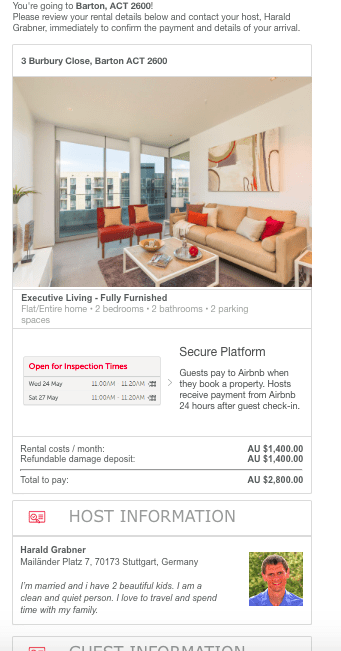**Descriptive Caption:**

This mobile screenshot depicts the rental details for an upcoming stay in Barton, ACT 2600, Australia. At the top, it confirms the destination as Barton, ACT 2600. Below this confirmation, there is a notice requesting the review of rental details and urging immediate contact with the host, Harald Grabner, to confirm payment and arrival details. 

The featured photograph showcases a modern and elegant living room, fully furnished for comfort and style. It includes a beige couch adorned with red, white, and beige pillows, two vibrant red chairs, and a stylish coffee table. The room is well-lit, thanks to a large window in the background, enhancing the contemporary ambiance of the space.

The property address is listed as "3 Burberry Close, Barton, ACT 2600". The listing highlights that it is an executive accommodation and comes fully furnished. A noticeable red box provides options for inspection times, signifying the availability for property inspection. 

To the right, it explains the secure payment process: guests pay via Airbnb at booking, and hosts receive payment 24 hours after guest check-in. The total rental cost is AU$2800. 

Further down, host information is displayed, featuring a profile picture of Harald Grabner, affirming him as the point of contact for any inquiries or issues. The entire screenshot is in color, enhancing the clarity and appeal of the information presented.